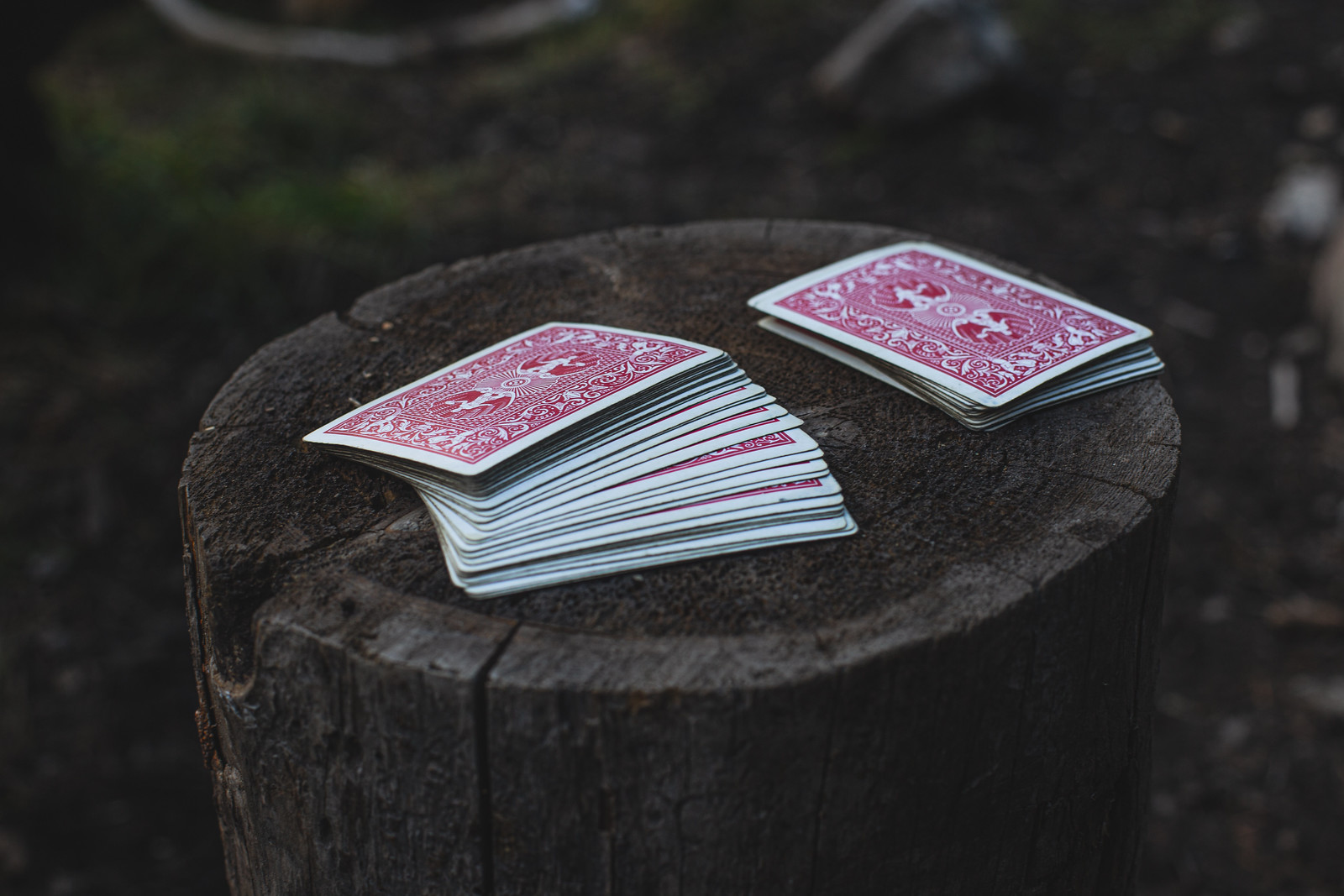In the center of the image, a wooden stump dominates the frame, showcasing its natural grayish and dark-toned cracks. The background is a deep black, drawing attention to the stump which stands out prominently in its surrounding. Flanking the stump on both sides are two stacks of playing cards. The cards are fanned out in a balanced manner, creating a mirror-like composition. The back of each card reveals an intricate red floral pattern with wavy lines, and they are bordered with white edges that provide a sharp contrast. Some cards appear slightly scattered around the stump, adding a dynamic element to the scene. The background remains out of focus, ensuring that the detailed textures of the wood and the ornate designs on the cards take center stage. On a closer look, the pattern on the cards seems to depict a figure standing in front of a lotus flower, adding an element of mystique and elegance.